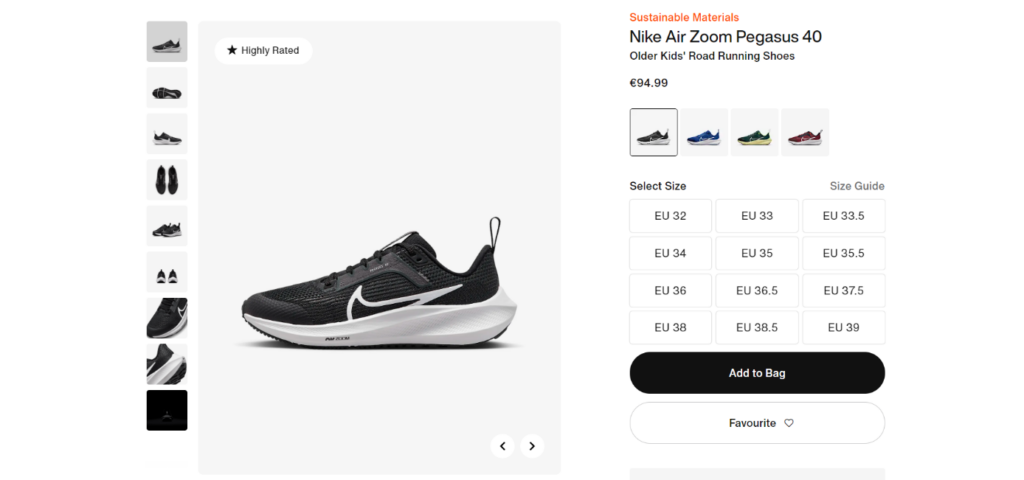This is a detailed screenshot from a shopping website displaying a black and white running shoe. On the left side of the page, nine vertical thumbnail photographs showcase various angles of the shoe. The main portion of the page is dominated by a large, detailed image of the running shoe, highlighted against a simple background. The shoe features a pristine white sole, a distinct white Nike swoosh on its side, and a predominantly black upper. A notable design element is a large loop located at the top of the heel area.

In the upper left-hand corner of the main image, a white oval box with a black star indicates that the shoe is "highly rated." To the right, in bold orange text, the phrase "sustainable materials" catches the eye, indicating an eco-friendly aspect of the product. Below this, in classic black text, the model name "Nike Air Zoom Pegasus 40" is displayed, specifically noting that these are "older kids road running shoes." The price is clearly marked at £94.99.

Below the main image, four horizontal thumbnails present the shoe in alternative colors: black, blue, yellow, and red, offering a glimpse at the variety available. User-friendly options such as different European sizes and a size guide are provided for convenience. At the bottom of the right side of the page, user interaction elements include buttons to "add to bag" or "favorite," enabling a straightforward shopping experience.